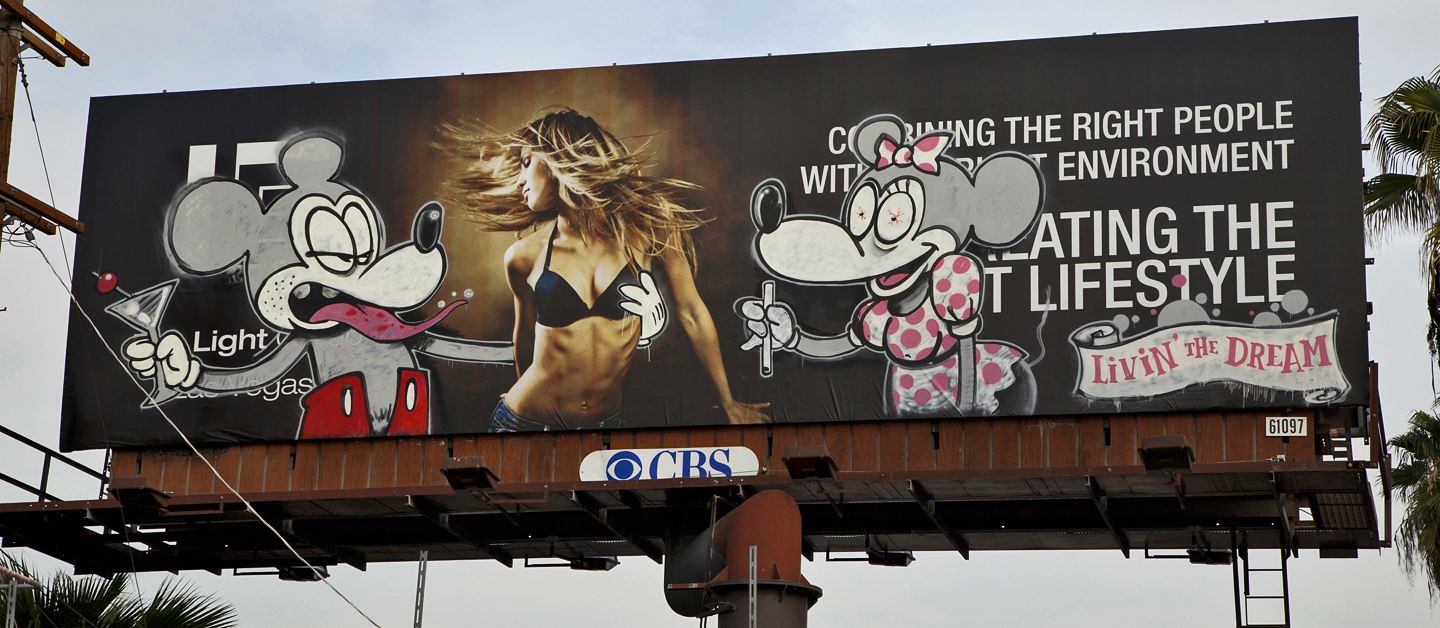The image showcases a large billboard viewed from below, emphasizing its imposing presence against the sky. The billboard originally features an advertisement with a model wearing a bikini top. To the right of the model, there's white text partially obscured by graffiti, vaguely discernible as conveying a message related to "lifestyle."

Superimposed on this billboard, graffiti artists have added two whimsical mice flanking the model. To the right of the model stands a female mouse adorned in a pink dress and a matching pink bow. Her eyes appear glazed over, adding a touch of surrealism to her expression. On the left side, a male mouse is depicted in brown pants, with a comically oversized red tongue hanging out of its mouth. This mouse, exuding a sense of playful mischief, holds a martini glass in its right, gloved hand while its left hand is suggestively caressing the model in the advertisement. The graffiti not only blends into the original billboard art but also infuses it with a layer of subversive street art character.